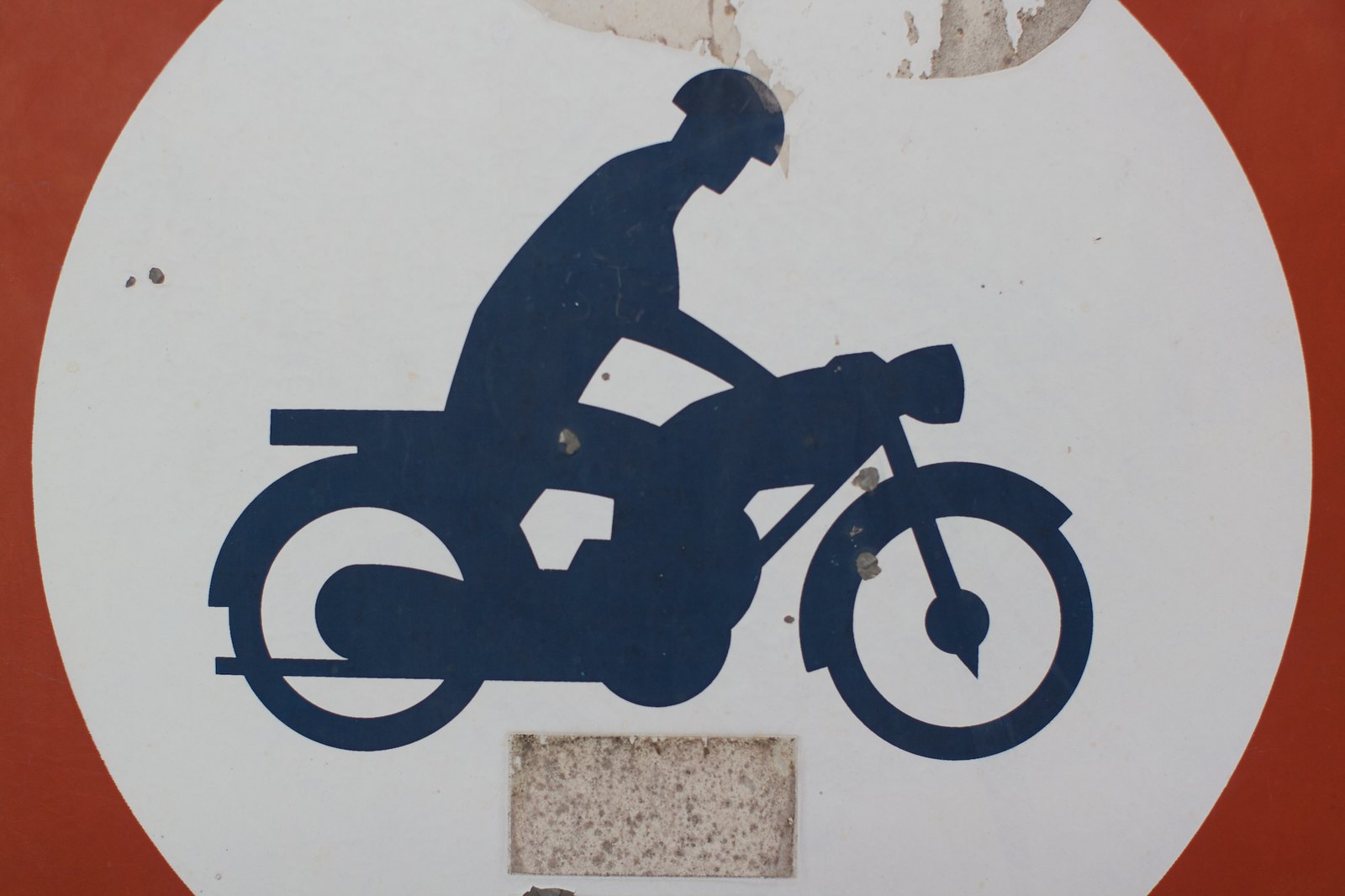The image shows a sign with a silhouette of a man riding a motorcycle. The background of the sign is a reddish-orange color, featuring a white circle in the center. Inside the white circle is the dark blue silhouette of the motorcyclist. The man is depicted in profile, bending over and gripping the handlebars, with his helmet clearly visible, though no facial features can be distinguished. Below the motorcycle, there is a rectangle that appears to expose the stone wall behind the sign, suggesting a cut-out or possibly an area where something was removed. The sign has some dirt or stain damage at the top, and there is adhesive residue suggesting that stickers might have been applied previously. The combination of colors and the visual prominence of the motorcyclist make the sign striking, despite its wear and tear.